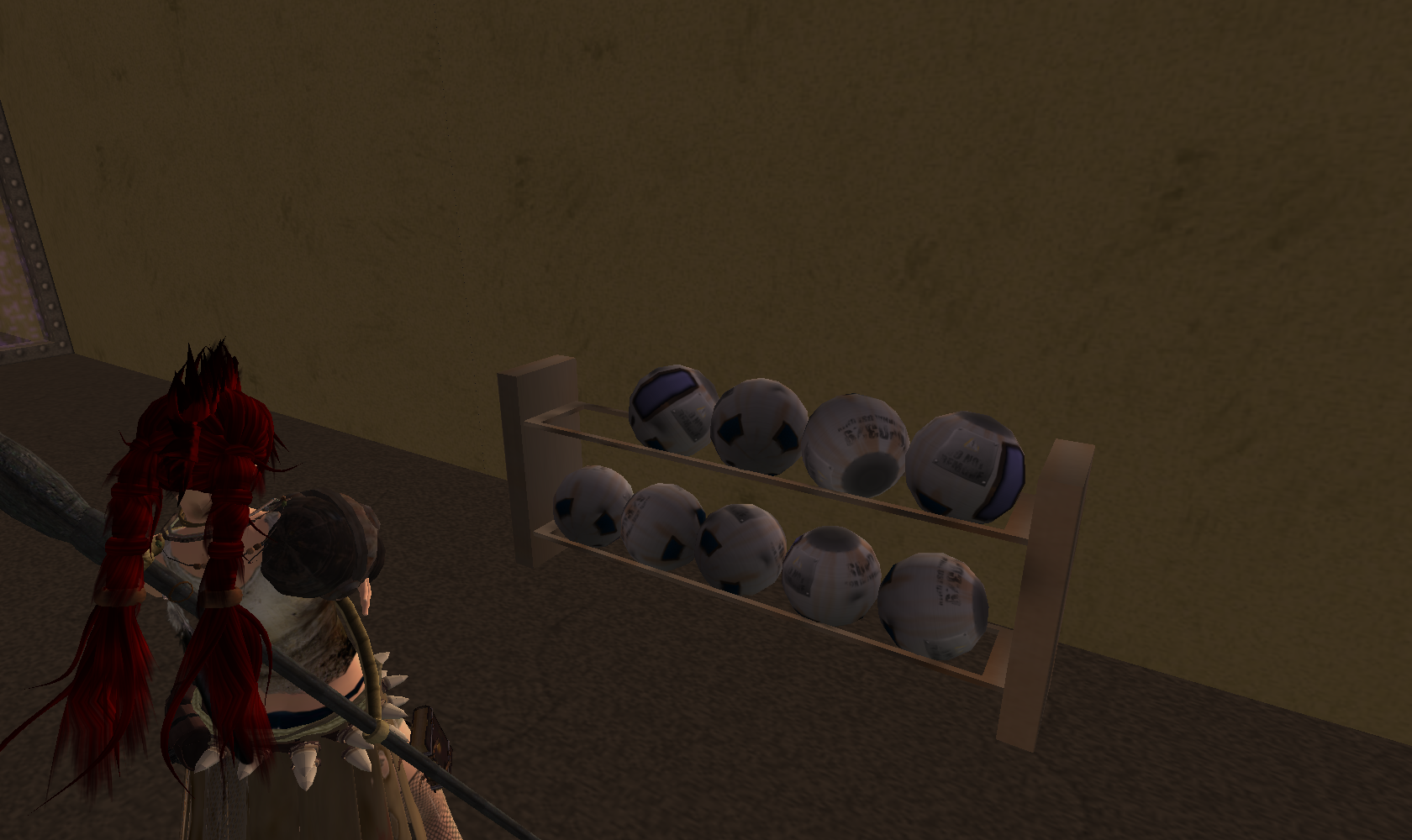The image appears to be a dark, computerized rendering of a room with a dark gray floor and a greenish-gray wall. Positioned against the wall is a wooden rack, possibly a crate, which stores several balls. The rack has two shelves, with the bottom shelf holding five volleyball-sized balls, while the top shelf contains four, suggesting one ball might be in use. Notably, to the left of the image, there is an indistinct object that looks like a red wig styled into braided pigtails, sitting on an unknown surface. This element adds a touch of ambiguity to the scene, possibly hinting at a little girl with red hair sitting in a chair and holding a baby doll, though this detail is less clear. Overall, the setting gives the impression of a space intended for storing athletic equipment, like a gym or an exercise facility.